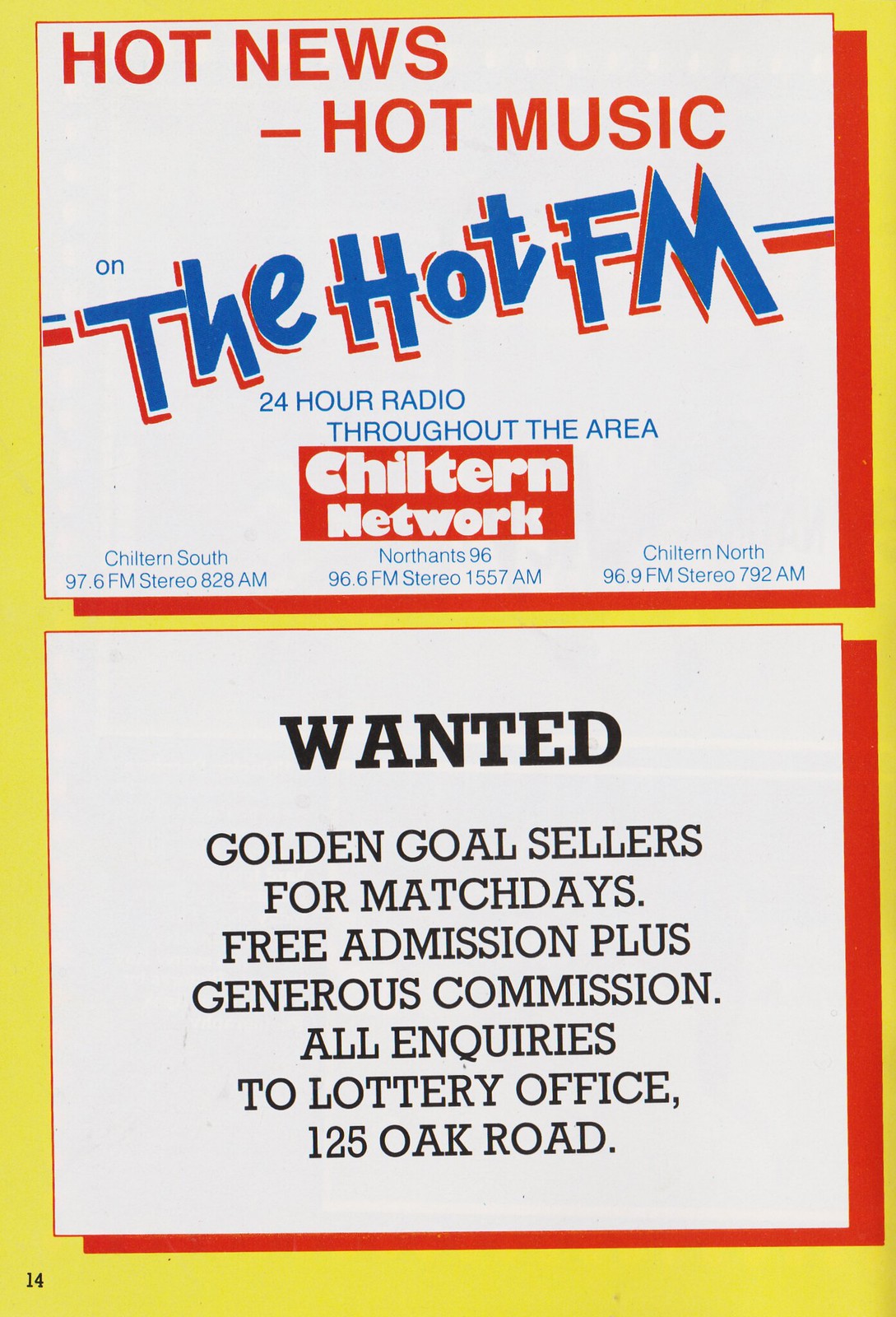The image is a rectangular, vintage print advertisement or business card, primarily featuring a yellow background with a red frame around two separate yet similarly styled ads, arranged vertically. The top section promotes a radio station and reads "Hot News - Hot Music on the Hot FM" in red and blue text. Directly below this, it notes, "24-hour radio throughout the area" in blue. Centered on the top ad, there's a logo for the Chiltern Network in bold white letters on a red horizontal rectangle. The ad then lists three specific radio stations: Chiltern South (97.6 FM stereo, 828 AM), North Ent (96.6 FM stereo, 1557 AM), and Chiltern North (96.9 FM stereo, 792 AM).

The bottom section of the image, set against a white background with a red frame, calls for "Wanted: Golden Goal Sellers for Match Days" in black text. It mentions free admission plus generous commissions and provides a contact address for inquiries: Lottery Office, 125 Oak Road. The overall design suggests a vintage style with spot coloring in blue, red, and yellow, typical of older print productions. The page is marked as page 14 on the bottom left corner.